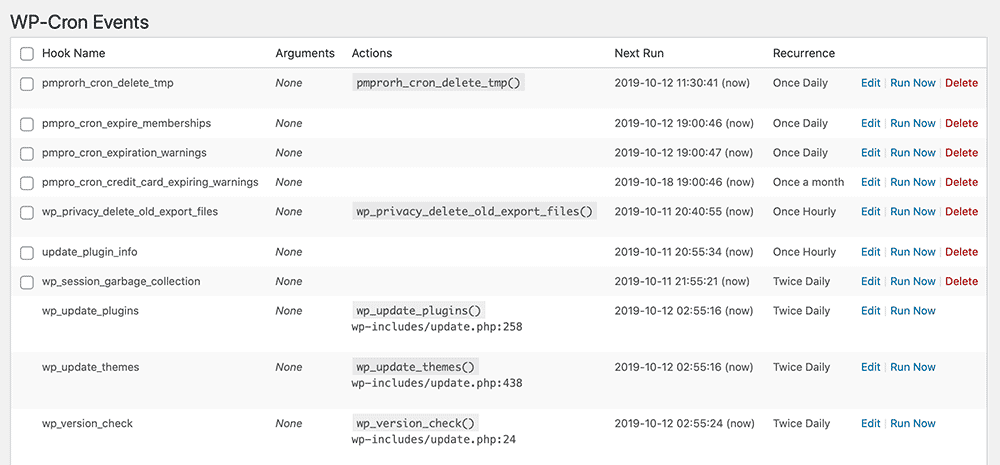The image features a webpage interface with a predominantly white background. At the top, there is a thick black or gray banner that extends downwards as a very thin border along the left and right sides. In the top left corner of the banner, the word "Dope" is displayed in black text. Next to it, the acronym "WP-Cron Events" is written, with "WP" and "E" in uppercase, "cron" in lowercase, and "V" in uppercase, followed by "ent" in lowercase, forming the word "V_ent".

Below the banner, the page alternates between white and gray backgrounds. At the top of the first section, a header row lists columns named "Hook Name," "Arguments," "Actions," "Next Run," and "Recurrence." Underneath, there are several rows filled with details.

On the left-hand side, there are checkboxes for each row, totaling eight in number. The sections under "Arguments" show "None" for the last three entries. The "Actions" column displays entries in the first, fifth, eighth, ninth, and tenth rows. The "Next Run" column indicates that all tasks are scheduled to run now. Under "Recurrence," the tasks are set to run at different intervals including "once daily," "once a month," "once hourly," "twice a day," and "twice daily."

Each row also features blue "Edit" and "Run Now" buttons, and the last three rows additionally contain a red "Delete" option on the far right-hand side.